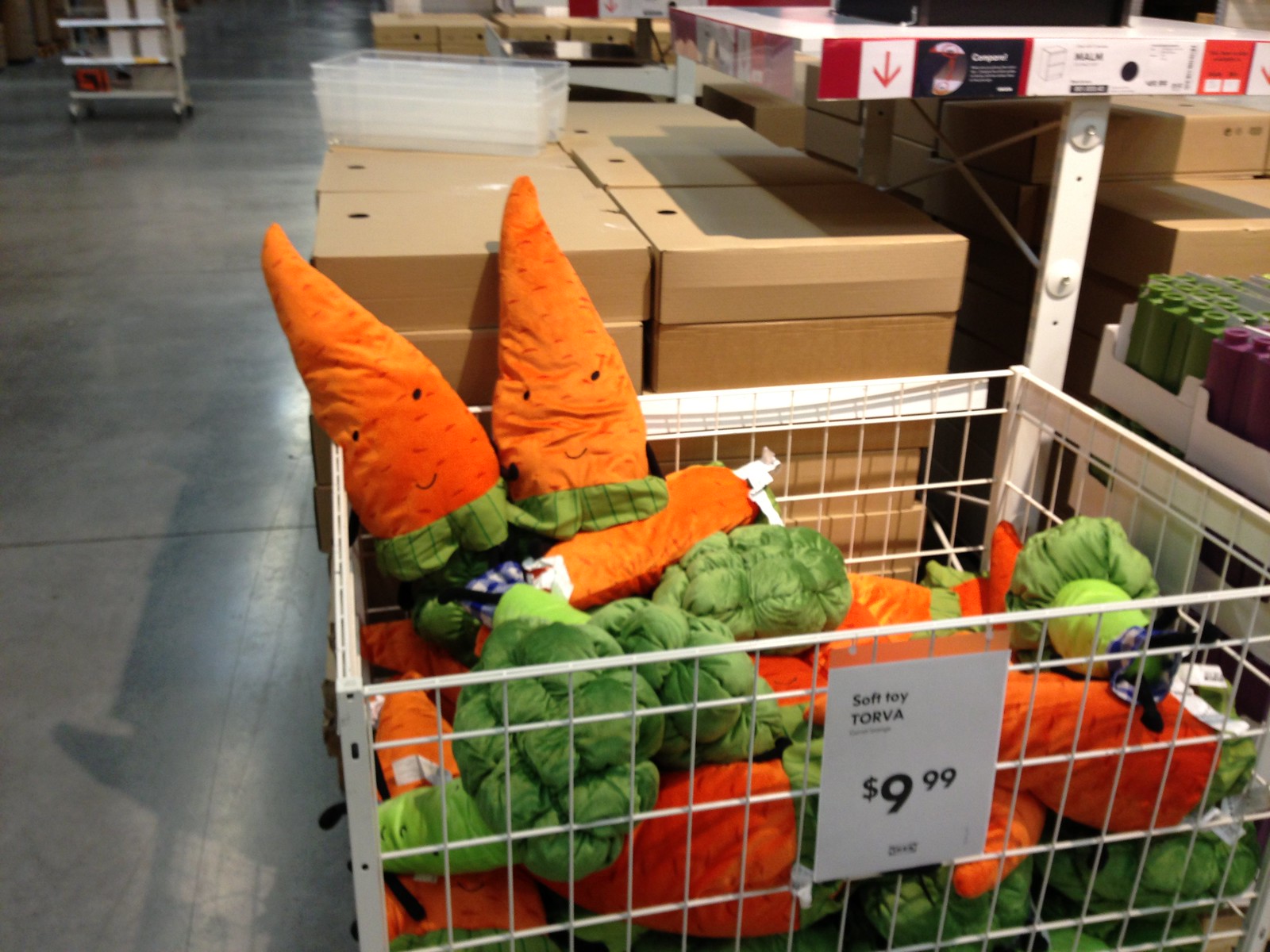The image showcases the inside of an Ikea store, featuring a variety of typical Ikea elements. Central to the scene is a white, see-through basket labeled "Soft Toy Torva" priced at $9.99. This basket contains multiple stuffed toys designed to look like carrots, with orange bodies, green leafy tops, and faces featuring black circular eyes and U-shaped mouths. The floor beneath appears to be industrial cement in a gray hue. Surrounding the basket, the store's decor includes flat-packed brown boxes, characteristic of Ikea's packaging, stacked behind it. To the right, there are white boxes holding green and purple painting containers. In the background, more flat-packed boxes are visible alongside a rolling cart, further emphasizing the store setting.